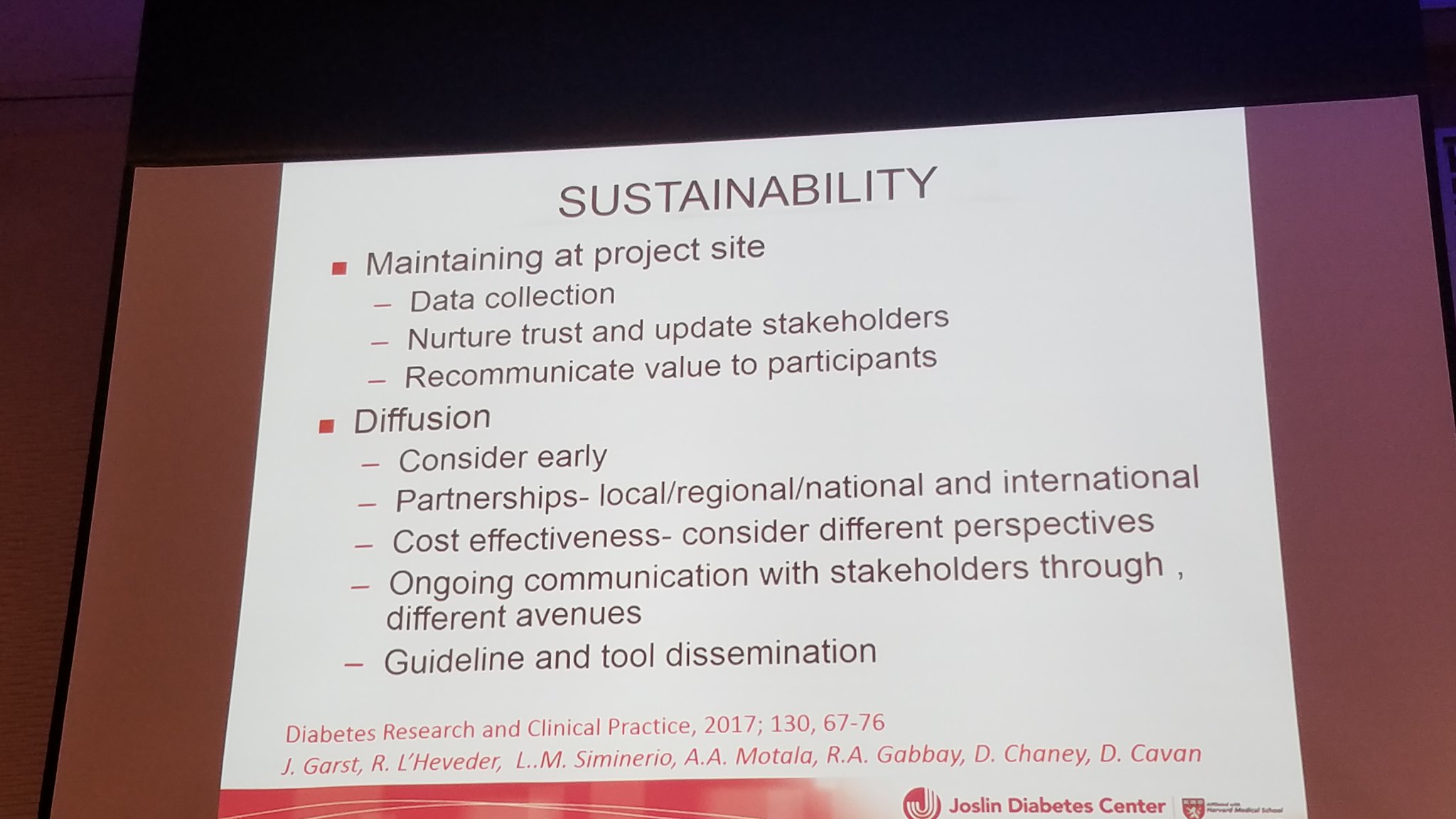The image depicts a PowerPoint slide projected onto a whiteboard, with a detailed layout focusing on sustainability. The background of the slide is primarily white, framed by a gradient border of rust and burgundy hues. The title of the presentation, emblazoned in all capital letters, reads "SUSTAINABILITY." Below the title, the slide is organized into two main sections, each introduced by a red square bullet point.

The first section, titled "Maintaining at Project Site," includes the following subpoints denoted by red dashes:
- Data Collection
- Nurture Trust and Update Stakeholders
- Recommunicate Value to Participants

The second section, titled "Diffusion," covers the following topics:
- Consider Early
- Partnership (Local/Regional/National/International)
- Cost Effectiveness

Additionally, there is intricate information on the need to consider different perspectives, facilitate ongoing communication with stakeholders through various channels, and disseminate guidelines and tools.

At the bottom of the slide, the source is credited to a publication or article related to diabetes research and clinical practice, with details including the publication date and time in red font against the white background.